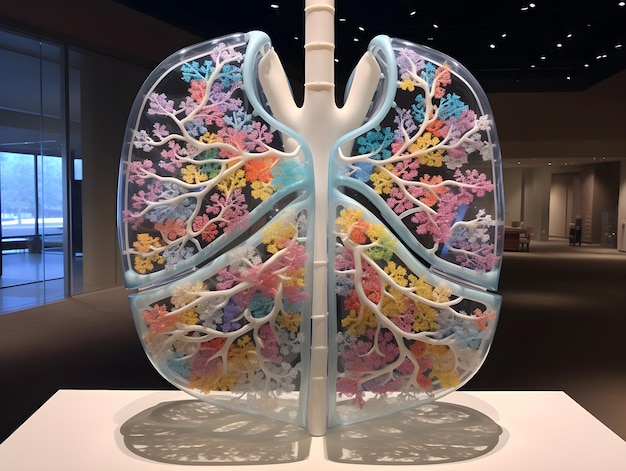The image depicts a detailed color photograph in landscape orientation, capturing an artistic 3D model of human lungs, prominently displayed on a white podium within a spacious, dimly-lit interior, possibly a museum or convention center. The model features a prominent white tube at the center, which branches into a W-shape forming two lobes at the top and two at the bottom. These branches are surrounded by a network of white vessels that likely represent bronchioles or blood vessels. The exterior of the lungs is encased in clear resin or plastic, giving it a glass-like appearance. The model is adorned with a vibrant array of colors—purple, blue, yellow, orange, green, and red—resembling coral or flowers intertwined with the white branches, symbolizing the inner workings and the left and right sides of the lungs. The overall structure creates a visually striking representation, mirrored perfectly down the center, with colorful floral patterns both on the top and bottom sections of the sculpture. The photograph also captures the reflection of this intricate model on the white table below. The background reveals other museum displays shrouded in darkness, punctuated by overhead lighting, and an open space extending into the distance, accentuating the grand scale of the room.